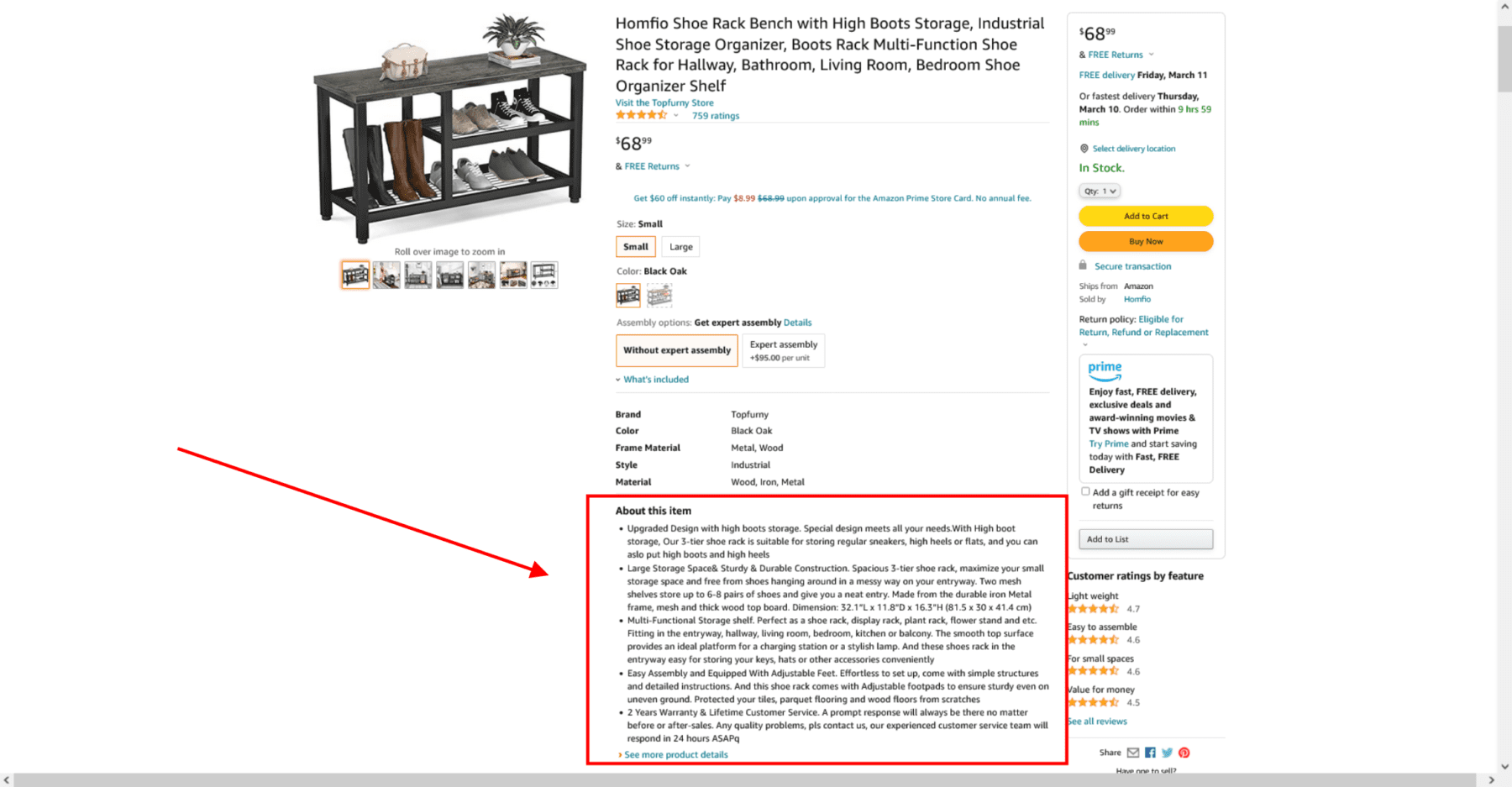This image showcases a multi-functional shelving bench designed for storing shoes. Situated in the upper left, a product image displays its compact design. The product information section is outlined in a red box, highlighted with a red arrow for emphasis. Although the text in this segment is slightly obscured, it is located at the lower center portion of the image. At the top center, the product title is prominently featured. Directly below the title, customer reviews indicate a favorable rating of four and a half stars. The product is priced at $68. 

Configuration options allow customization for size and color; currently, 'small' and 'black oak' are selected. Detailed specifics of the product—covering aspects such as brand, color, frame material, style, and material—are outlined beneath these options. The "About This Item" section, marked for easy visibility, lists five key bullet points that further describe the product features and benefits.